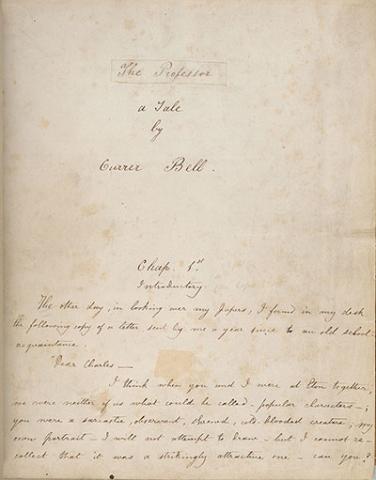The image features a single brown, aged, and stained sheet of paper that has a vintage look, akin to old newspaper parchment. The text is handwritten in calligraphy, making it difficult to decipher. The title at the top reads "The Professor, a Tale by Gore Bell." Further down, the paper reveals a section labeled "Chapter 1, Introduction." Although the paragraph below this heading starts with "the other day,” the rest of the text on this page is unclear due to the ornate calligraphic style. The entire image comprises just this piece of paper, without any additional objects or elements. The overall coloration consists of various shades of brown, reinforcing its old, weathered appearance.